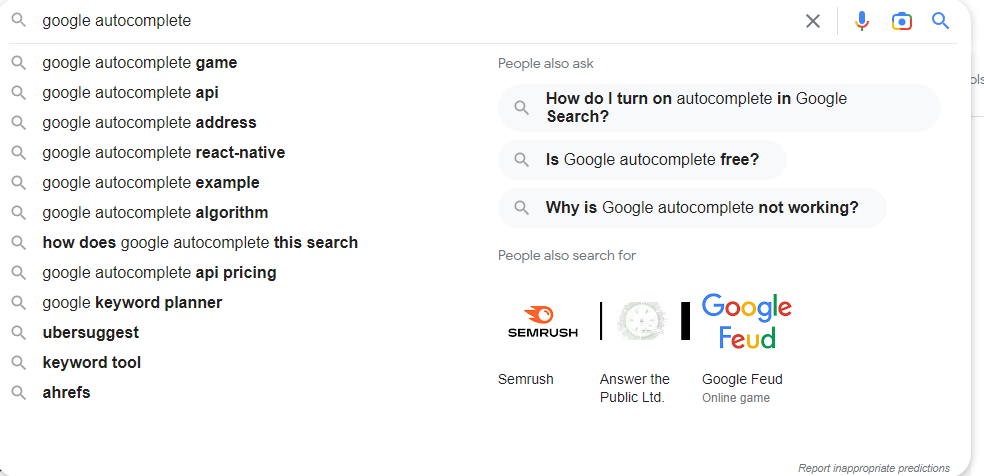This screenshot captures a Google search results page centered around the query "Google autocomplete." The left side of the image prominently displays the search term "Google autocomplete," followed by a list of autocomplete suggestions that include: 
1. Google autocomplete game 
2. Google autocomplete API 
3. Google autocomplete address 
4. Google autocomplete react native 
5. Google autocomplete example 
6. Google autocomplete algorithm 
7. How does Google autocomplete the search 
8. Google autocomplete API pricing 
9. Google keyword planner 
10. Ubersuggest 
11. Keyword Tool 
12. Ahrefs 

The suggestions appear in a somewhat darker font than the rest of the text, making them stand out.

On the right side of the screenshot, the section titled "People Also Ask" lists three common questions related to Google autocomplete: 
1. How do I turn on autocomplete in Google search? 
2. Is Google autocomplete free? 
3. Why is Google autocomplete not working?

Beneath this segment is another section titled "People Also Search For," which includes three items: 
1. SEMrush 
2. Answer the Public Ltd 
3. Google Feud, followed by "Google Feud online game"

At the very bottom right corner of the screenshot, there is a note in small text that reads "Report inappropriate predictions."